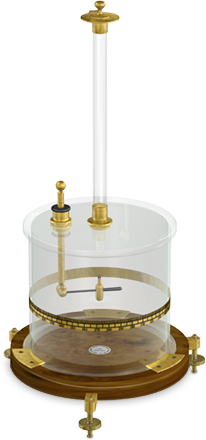The image showcases an antique weather device with an elegant, intricate design. The object features a brown base, which appears to be made of either wood or metal, adorned with gold hardware and brass hinges. Supporting the base are three or four gold legs. Resting atop the base is a clear glass dome, held securely by gold hardware, with an intricate gold band encircling its middle. Inside this dome, a central glass tube extends vertically through the dome and rises approximately double its height. Topping this glass tube is a gold umbrella-shaped cap. To the left of the central tube, a smaller gold-armed instrument also pierces the top of the glass dome. This smaller instrument is mounted to the base at the center and contributes to the ornate design encircling the glass dome. The careful craftsmanship and materials suggest it is an antique observational or meteorological instrument, though there is no lettering or additional context to confirm its specific use.